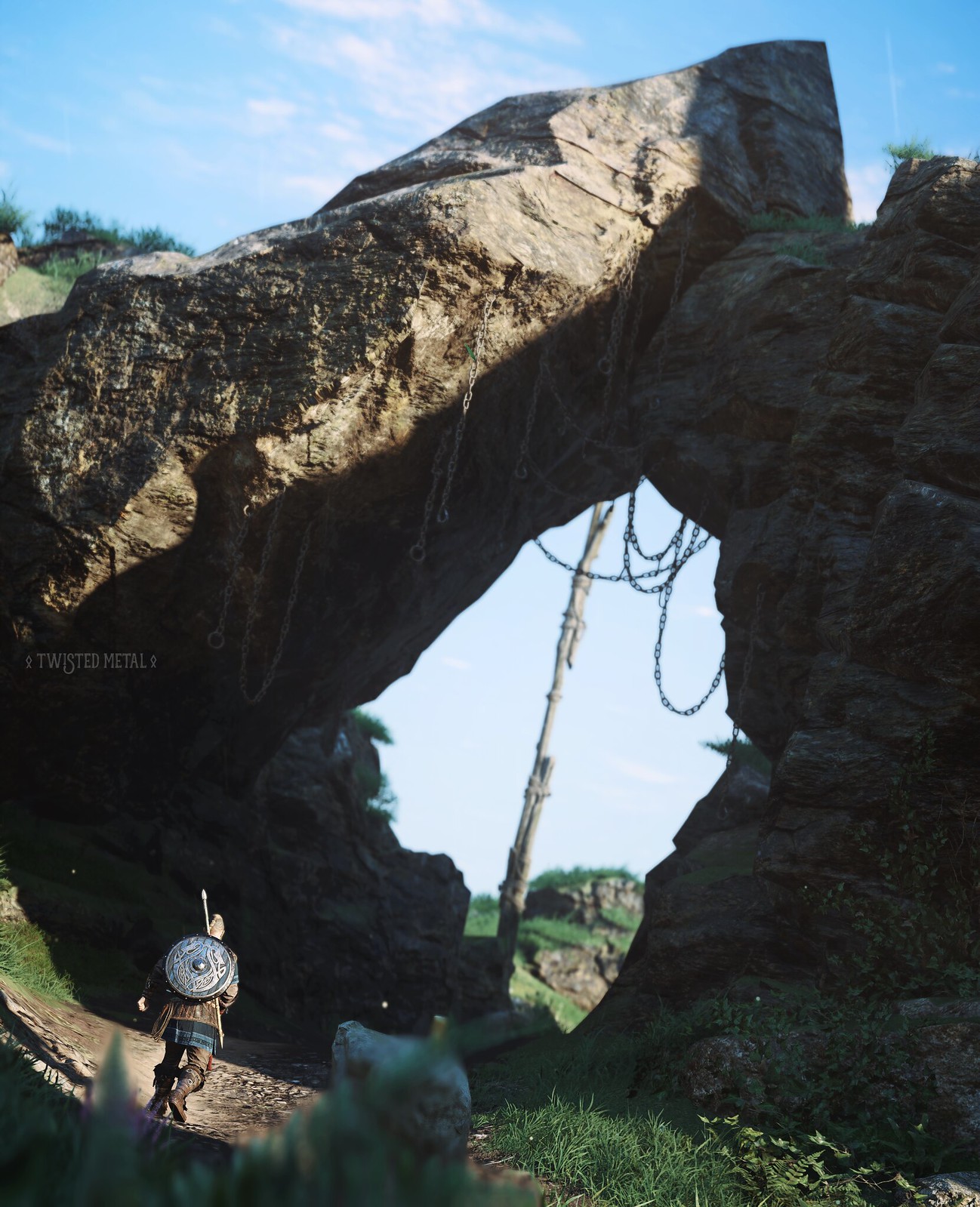Under a clear blue sky with wispy white clouds, an ultra-realistic scene, seemingly from a video game possibly titled "Twisted Metal," unfolds. The focal point is a prominent natural stone archway adorned with hanging chains. To the left of the archway, verdant green grass and trees dot the landscape, adding a touch of nature amidst the rugged terrain.

In the bottom left corner, a warrior clad in ornate armor is depicted. The circular, intricately carved shield on his back, along with his topknot and thigh-length tunic, convey an ancient, almost mythic aura, reminiscent of Scottish warriors. He is striding forward in long brown boots, holding a spear that extends past his head. This dynamic character is poised to walk under the enigmatic archway. The watermark "Twisted Metal" can be seen on the left-hand side of the image, further suggesting the video game context.